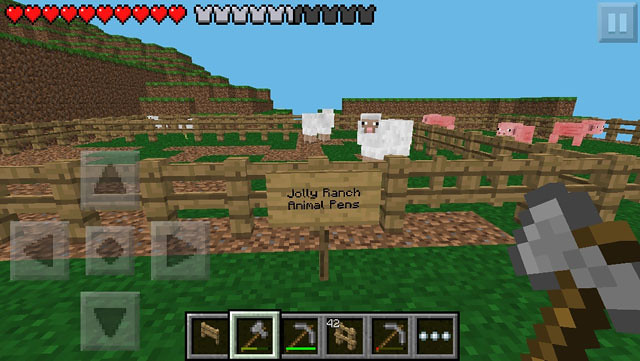This is a screenshot from a blocky, pixelated computer game, reminiscent of Minecraft but not as detailed. Central to the image is a light brown, rectangular wooden sign with black text reading "Jolly Ranch Animal Pens." The scene features various animal pens made of light brown fencing with dark accents. Inside the middle pen, there are block-like sheep with white and gray colors, dark brown faces, and small, detailed eyes and mouths. To the right, another pen contains four pink pixelated pigs with red splotches and similarly detailed eyes.

The foreground showcases blocky green grass and soil, with the background depicting a sky gradient from light blue above to darker shades below. There's also a distant mountain crafted from dark brown blocks, transitioning to a mix of light and dark green at the peak.

Across the top left, a row of ten red hearts indicates player health, while adjacent, a series of icons resembling gray t-shirts displays damage or armor status, with the first five icons white, the next half white, half black, and the remaining four black. In the upper right corner, an icon resembling an electrical outlet or a d-pad is visible, featuring black directional arrows on a gray background.

The lower part of the screen reveals various game interface elements including hero and tool icons. The bottom center has six squares, each containing different game icons: items like fences, an axe, and a pickaxe, with health bars and quantities displayed. The player's current tool, a pixelated axe with multiple shades of gray and a wooden handle, is prominently visible. The vibrant, blocky aesthetic of the game emphasizes an old-school charm, enhancing the farm and animal theme of the scene.